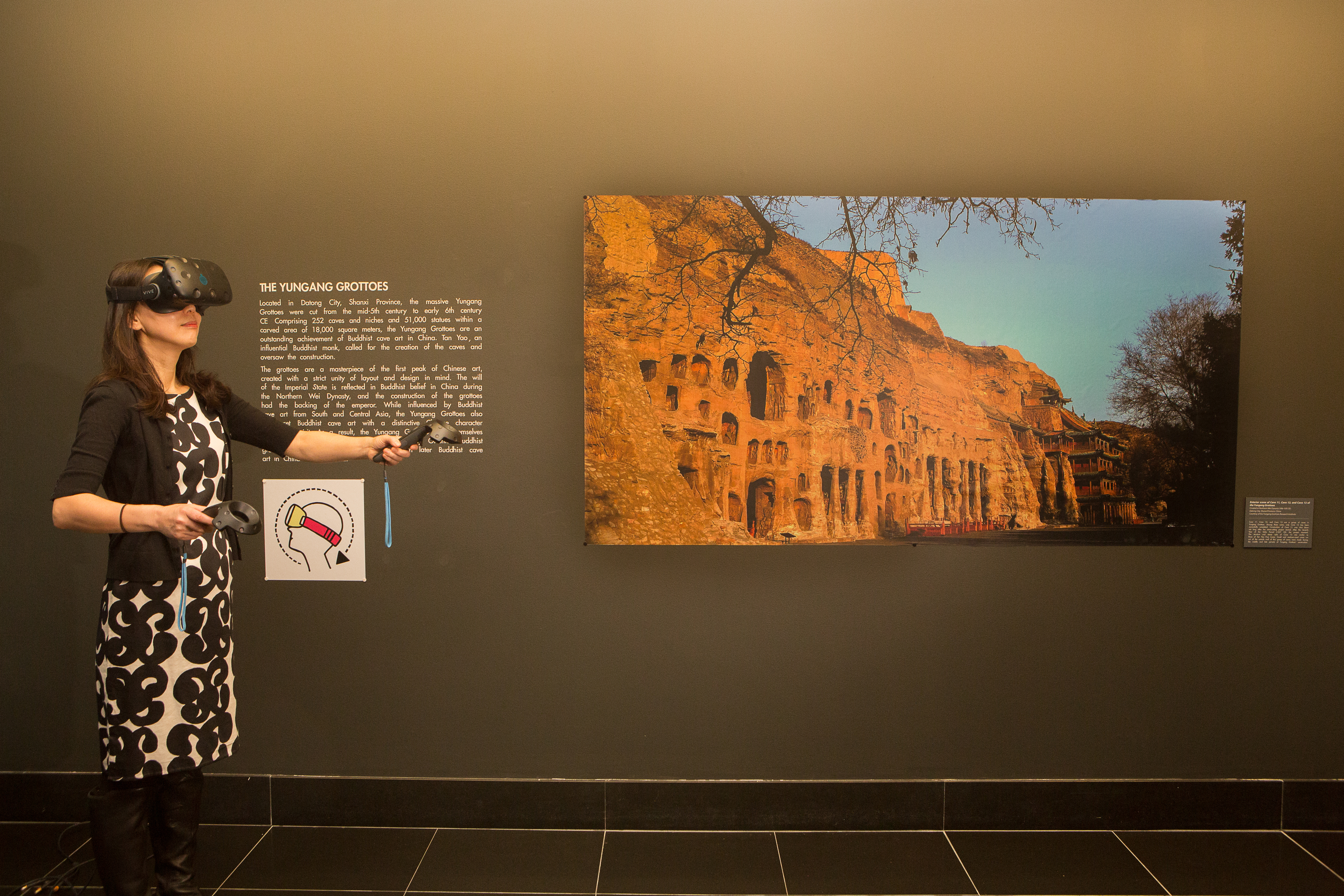In the image, a white woman with long brown hair is seen interacting with a virtual reality exhibit in what appears to be a museum. She is wearing a black VR headset with controllers in both hands. Dressed in a black and white swirl-patterned dress paired with a black suit jacket and black boots, she stands on the left side of the picture, facing right, her left arm extended straight out and her right arm slightly forward. Behind her is a brown wall featuring an image of the historical Jiangang Grottoes, located in Dalang city, Shanxi province, China. The background also includes descriptive text about the site and a stone wall that looks ancient. The upper part of the wall is dark green while the floor is a matching dark green or black tile, bordered by a trim of the same color. The scene suggests an intriguing blend of ancient history and modern technology, inviting museum-goers to immerse themselves in a virtual exploration of the grottoes.